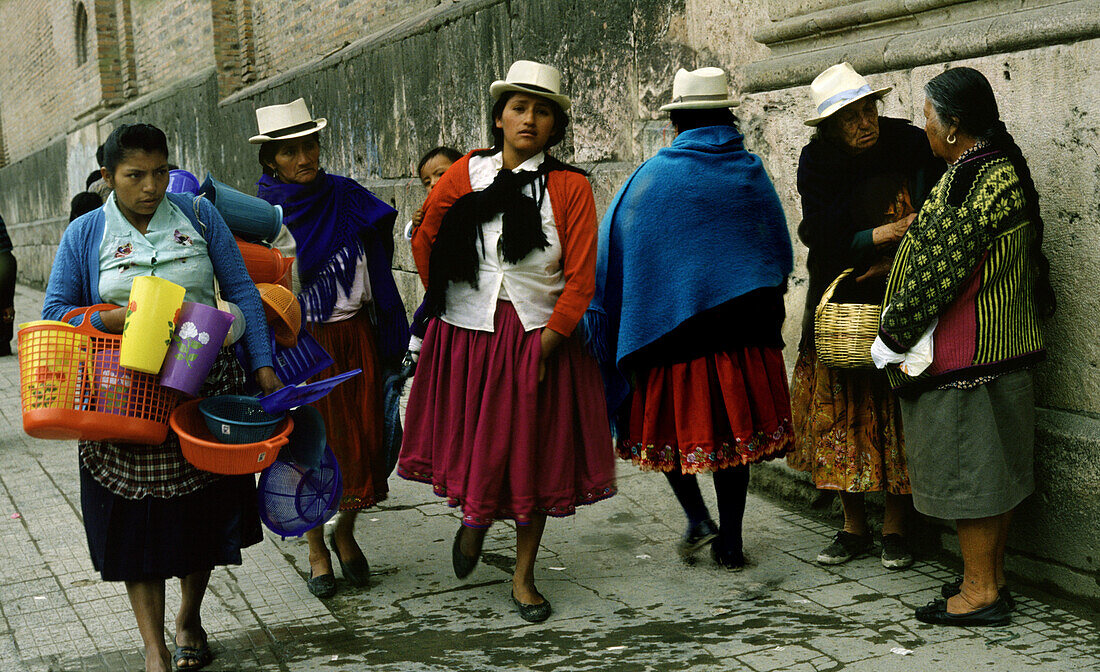In this lively street scene, a group of women, likely in a Latin American or South American country, walk down a gray sidewalk in front of a gray wall. The women, who appear to be of darker skin tones, are dressed in colorful skirts and flat-bottomed shoes similar to ballerina flats. Many of them wear white hats with black sashes or ribbon bands, which resemble fedoras, and have their hair pulled back into long braids. 

On the right side of the image, two older women stand off to the side, engaged in conversation. The older of the two, holding a wicker basket, wears a distinctive hat seen on several others in the image. The younger woman beside her has a long braid and a hoop earring. Moving leftward, another woman in a white hat, red skirt, and blue shawl over her shoulders walks away from the photographer.

To her left, a prominent woman facing the camera stands out in a white shirt, orange sweater, and a reddish-magenta skirt. A child peeks over her shoulder as she carries them on her back. Nearby, another woman, similarly attired in a white hat and blue shawl, dons a strikingly similar red skirt.

On the far left, a woman laden with multiple pitchers, baskets, and pots walks towards the photographer. Her blue sweater, white shirt, and blue skirt with an apron complete her look. Her hands and back are visibly full, suggesting she might be selling these items.

The overall scene captures the cultural essence and daily life of these women, showcasing their traditional attire and communal interactions.